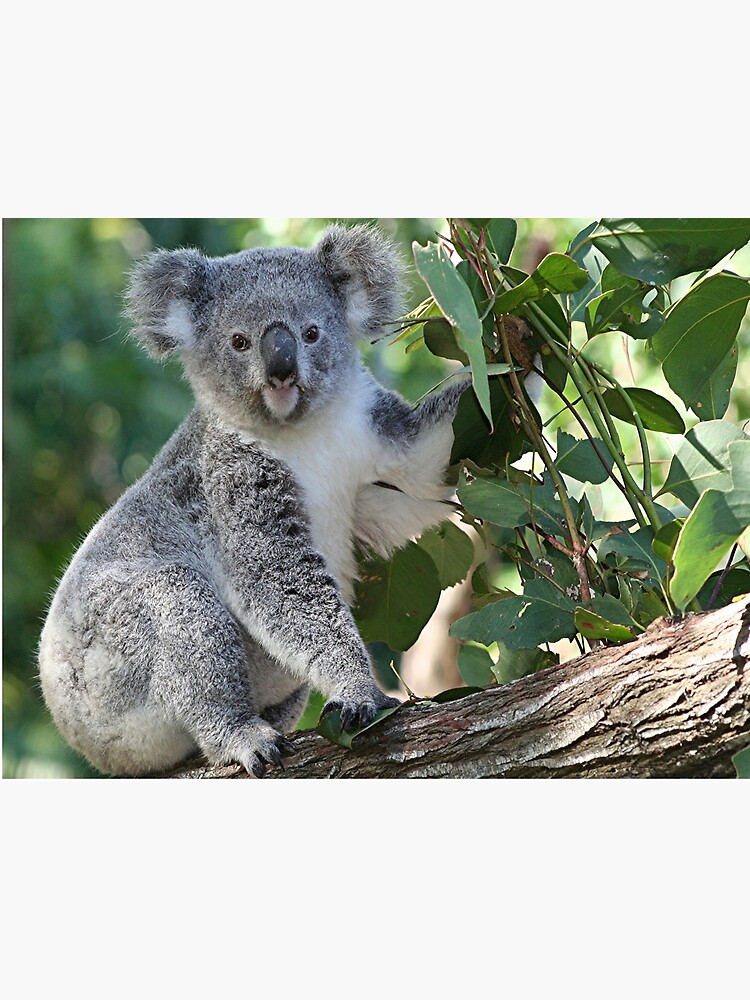In this beautifully lit daytime outdoor scene, a cute koala bear takes center stage, perched serenely on a large branch. The background is an inviting blur of lush greenery, hinting at a forest filled with trees and foliage. The koala, characterized by its soft gray fur with white accents, has a distinct little black nose and expressive black eyes. It grasps a handful of young eucalyptus leaves, possibly about to munch on them. With one forepaw gripping the branch and its curious gaze directed towards the camera, the koala exudes a peaceful and content demeanor amidst an abundance of natural light and verdant surroundings.